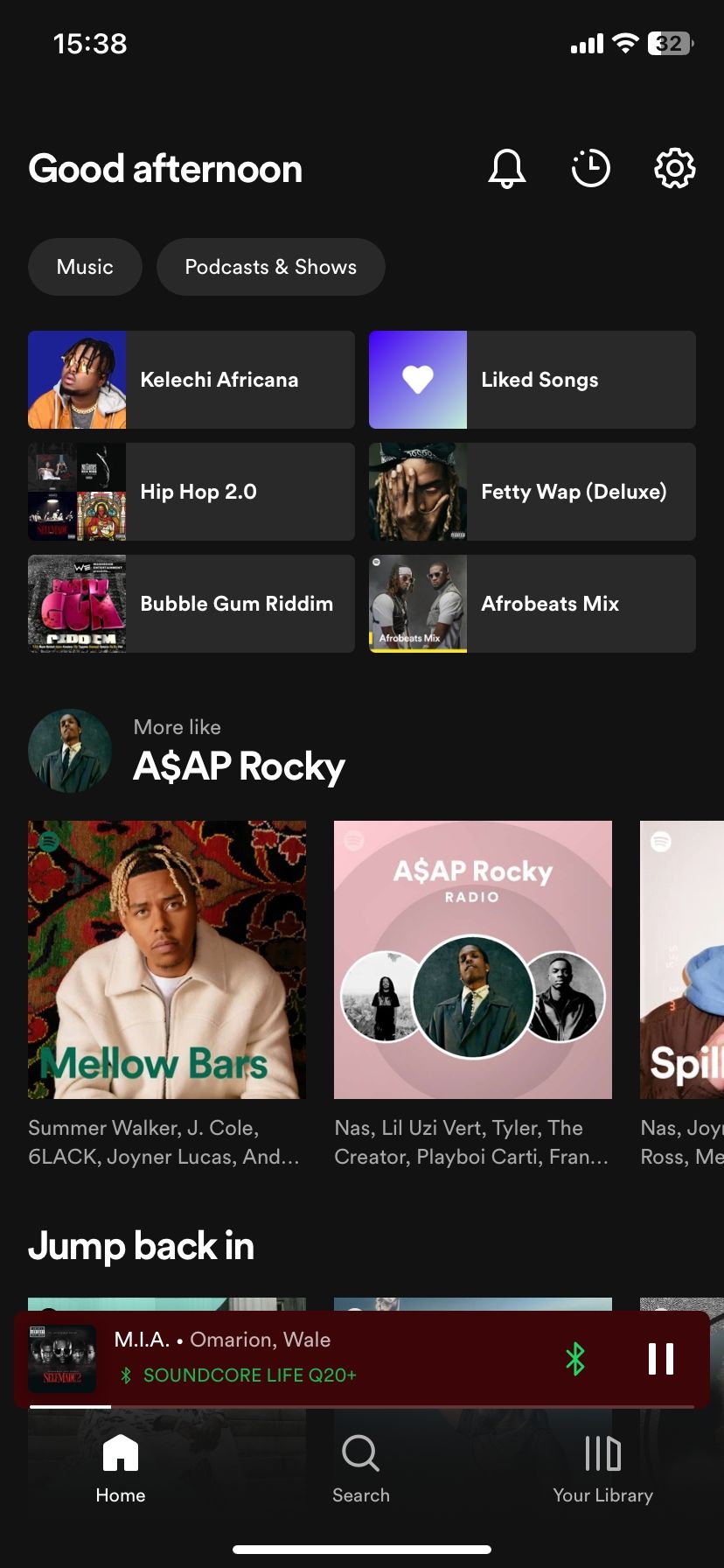This is a detailed screenshot of someone's music streaming page, showcasing various interface elements and musical content. At the very top, the time is displayed as 15:38, accompanied by indicators on the right: the service bars are fully filled, the WiFi signal is strong, and the battery level is at 32%. Beneath this header, a greeting reads "Good Afternoon." To its right, there are icons: a bell with notification dots at the 10 and 11 positions, an analog clock symbol with hands pointing at 12 and 3, and a settings gear icon.

The main content area introduces sections for "Music" and "Podcasts and Shows," with thumbnail images next to each category for easier navigation. The featured playlists and albums include "Caliche Africana," "Hip Hop 2.0," and "Bubblegum Rhydium." Adjacent to this list are "Liked Songs," "Fetty Wap (Deluxe)," and "Afro Beats Mix."

Further down, a section labeled "More like A$AP Rocky" appears, featuring a circular image of a man standing in the middle. This is followed by three album covers under the title "Mellow Mars A$AP Rocky Radio." 

Continuing to scroll, there is a "Jump back in" section, indicating recent listening activity with "M.I.A. Amarion Whale" currently being played.

The navigation bar at the bottom of the screen includes three main icons: a home symbol on the left, a search icon in the middle, and a "Your Library" option on the right.